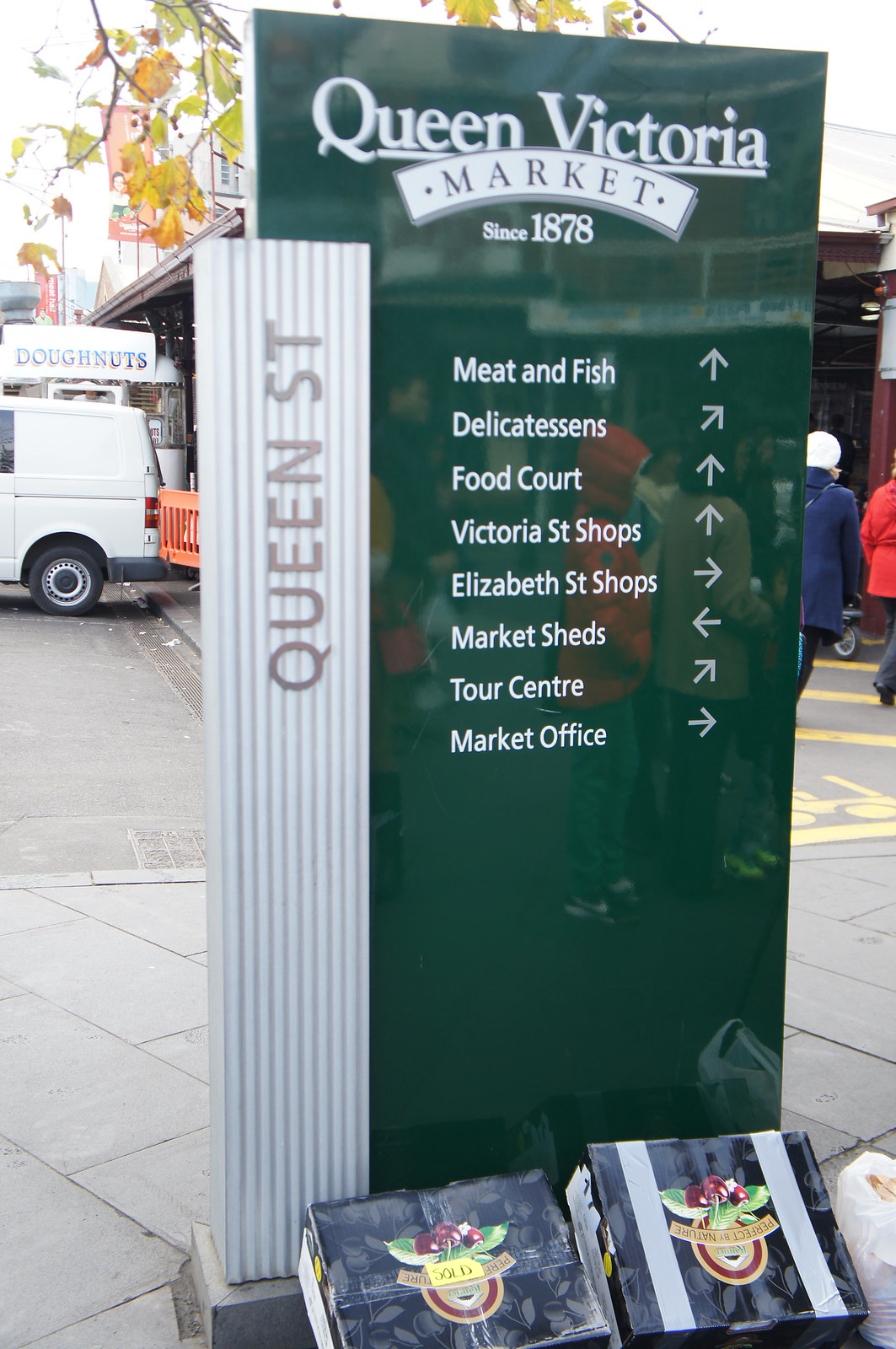An outdoor directory sign for the Queen Victoria Market, established in 1878, stands prominently. The highly reflective, green, rectangular pillar features a protuberance on its left side, labeled "Queen Street." At the top of the sign, in white font, are the words "Queen Victoria Market since 1878." Below, a list of various departments and shops is displayed alongside directional arrows: "Meat and Fish" (upwards), "Delicatessens" (top right), "Food Court," "Victoria Street Shops," and "Elizabeth Street Shops" (all upwards), "Market Sheds" (left), "Tour Center," and "Market Office." The directory sign is shiny enough to reflect people nearby, indicating its metallic surface. Surrounding the base of the sign are boxes and bags, including some cherry boxes labeled "perfect by nature," one with a "sold" sticker. In the vicinity, additional signage, such as one for "Donuts" and a white van, are visible, along with several market-goers.